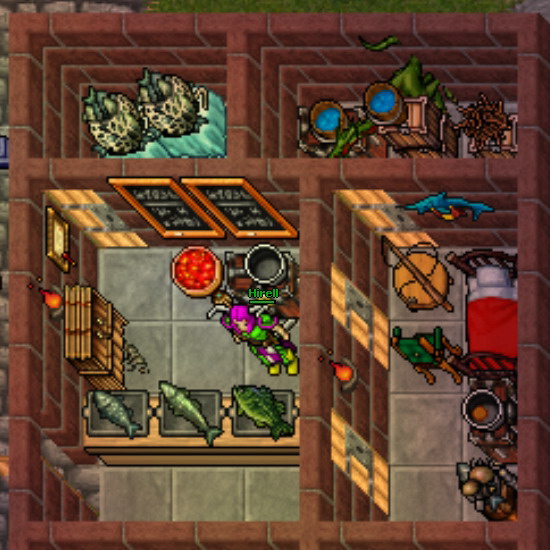The screenshot from a pixelated video game, reminiscent of a 32-bit design similar to Stardew Valley but of slightly lower quality, presents a top-down view of a brick building divided into four rooms. Starting from the bottom left, we are inside what appears to be a fish store. This room has a wooden display featuring three metallic trays, each holding a fish: a light blue fish, a light green fish, and a larger dark green fish. The shopkeeper standing nearby is named Hirel, identifiable by their pink hair and green warrior outfit, complete with lighter green shoes and pink-rimmed clothing. The shop walls are adorned with two wooden-rimmed blackboards and a candle-like flame above a cupboard. There's a bowl of red fruits, possibly tomatoes, and a cooking pot behind Hirel.

Adjacent to the shop on the right is a smaller rectangular room with a wooden door. Inside, there's a chair on the left side with a fishing rod draped over it, a large bag on the floor, and a cooking station with a big pot containing what appears to be a hamburger. A wooden bed with a red duvet and a white pillow is positioned beside a small wall ornament, possibly a statue.

Moving further right, an adjacent small room features several water buckets, boxes, and a few plants. To the left of this storage room, two grotesque frog-like creatures (referred to as large "fishies") can be seen.

Lastly, alongside the room with the fish display, there is a bedroom with a red bed and a white pillow, further adding to the essential homely elements of the game. The entire building is constructed from bricks, and the floor is paved with large square stone-grey tiles, further adding to the vintage gaming aesthetic.